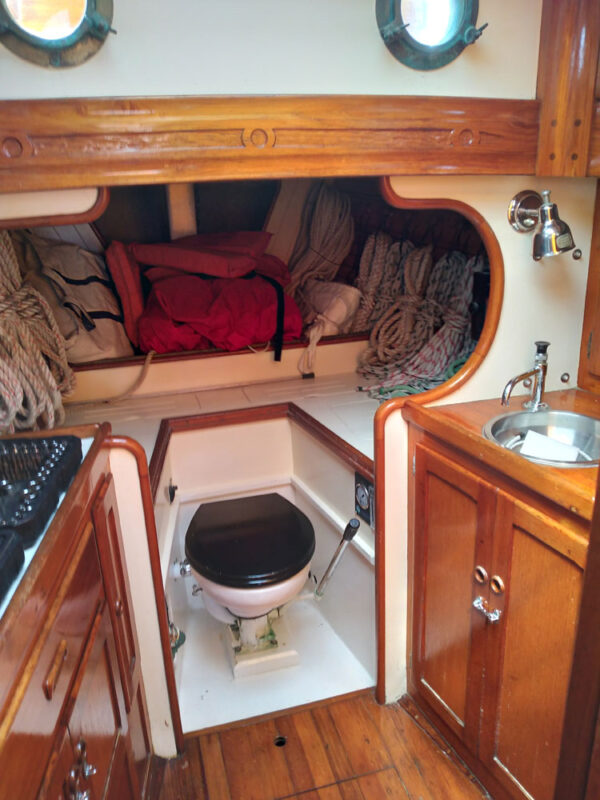The image depicts a compact bathroom on what appears to be a boat, likely a narrowboat or similar vessel. The layout is unusually tight and linear, characteristic of maritime design. Central to the scene is a toilet with a black seat, nestled into a recessed section of the wall that doubles as a makeshift storage area. This alcove above the toilet contains various boating necessities like ropes, bags, and life vests, suggesting it's a functional space for a crew. Flanking the toilet on either side are wooden cabinets, adding to the storage capabilities of the confined area. 

On the right side, there is a small, circular, stainless steel sink with a moveable tap and a light fixture positioned above it. The cabin is adorned with wooden cabinetry and white walls, and the floor is made of wood, enhancing the nautical aesthetic. Above the setup are two small, round porthole windows that seem to let in minimal natural light, possibly indicating the photo was taken at night. The overall color scheme contrasts the natural wood tones with white, further emphasizing the maritime theme. Additional elements include a lever, likely the flush mechanism for the toilet, and a peculiar gauge, hinting at the specialized nature of the equipment within the space.